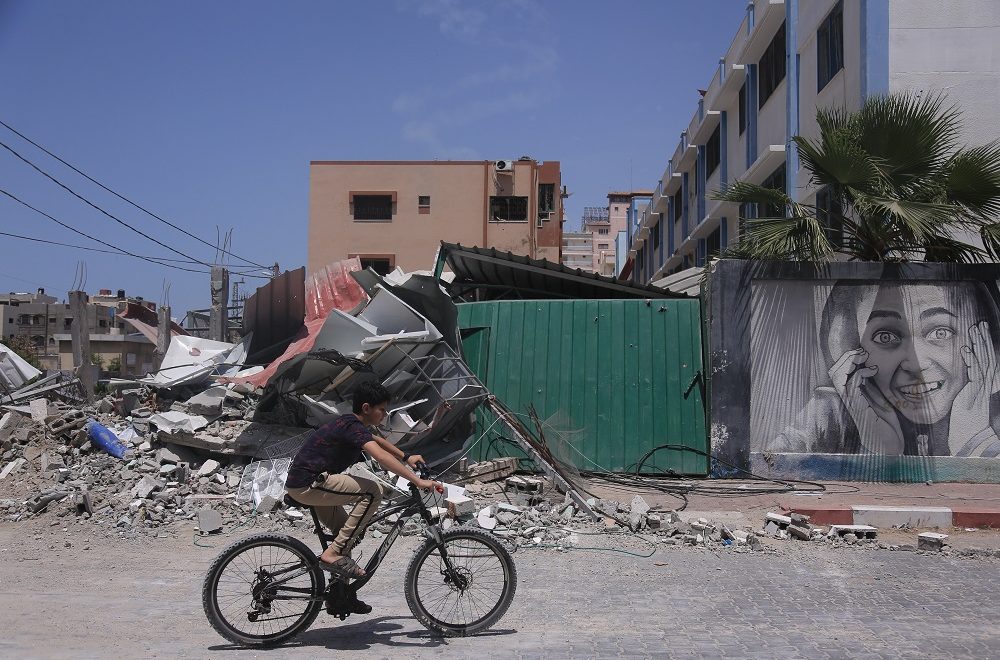In this detailed landscape-oriented image, a young boy with black hair is riding a gray and black bicycle towards the right side of the frame. He is dressed in a black t-shirt, tan pants with a black line down the side, and black sandals, and he is wearing a black wrist device on his left wrist. The backdrop is a stark, rundown urban area, appearing as if recently devastated, possibly even bombed. The sky above is mostly clear with a few white clouds scattered across the blue expanse. 

The shattered concrete buildings behind the boy show diverse shapes and sizes, with exposed wiring and twisted metal, contributing to the chaotic scene. Piles of grey rubble, varying from dark to light shades, dominate the ground. A conspicuous, dark green dumpster, approximately five feet tall with its lid half-opened, adds to the desolate atmosphere. Among the ruins, a mural painted in gray depicts a woman with a surprised expression, holding her hands to her cheeks. In the distant background, intact structures include a large tan building and a blue-and-white three-story apartment complex. The poignant artwork and the juxtaposition of destruction foreground the resilience and innocence of the child navigating through this environment on his bicycle.